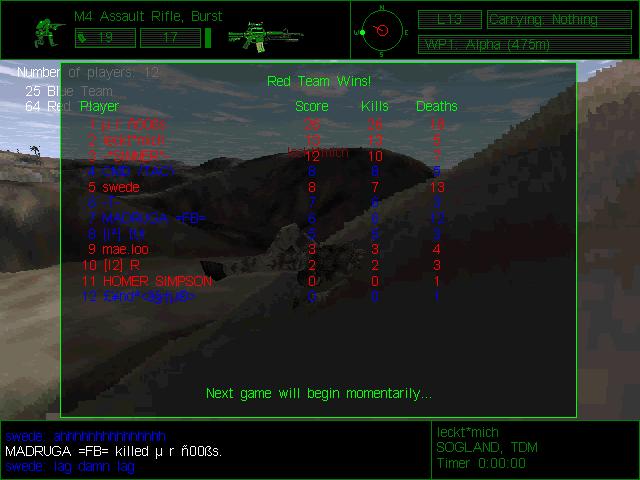This detailed caption combines the key elements shared across the three descriptions:

The image is a screenshot from a multiplayer shooting video game. Dominating the screen is the announcement "Red Team Wins" displayed prominently in the center. Directly below, there are columns listing players along with their scores, kills, and deaths, with these stats written in various colors: player scores in red, kills and deaths in green, and additional details in blue. The top-left corner shows a player stat menu with the labels "M4 Assault Rifle Burst" alongside icons of a soldier and an assault rifle, as well as numerical indicators likely representing remaining ammunition. At the bottom, a message reads "Next Game will begin momentarily," and towards the bottom-right corner, there's some unclear text in blue and white and the words "Select Michigan Saugland Tom Timer Zero." The background of the screen displays a scenic view of hills, indicating it's part of the game's environment. The overall color palette includes green, red, blue, and dark tones from the backdrop.